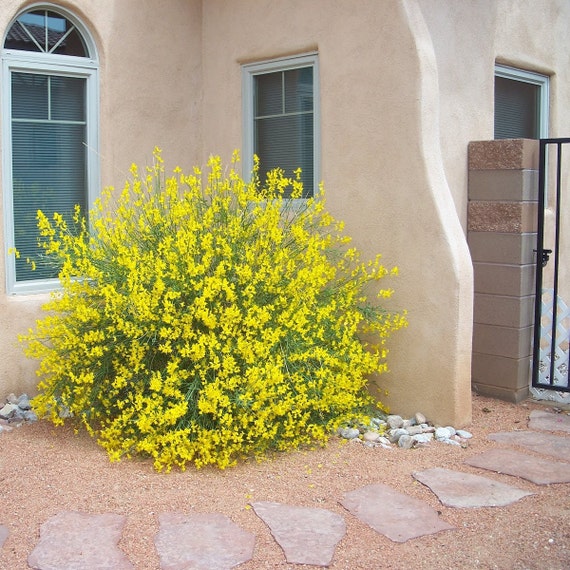The image depicts a desert-like house, possibly an Airbnb, characterized by a stone exterior and sandy gravel ground. At the corner of the house stands a tall, green shrub nearly five feet in height, identified as a Spanish bloom or broom plant, adorned with numerous yellow flowers. The house features a window on one side and a smaller window on the right corner, contributing to its desert aesthetic. In the foreground, a pathway composed of pink stepping stones leads to the right, culminating at a black gate. The scene is devoid of people, focusing solely on the house's unique architectural style and the vibrant desert flora. Various colors are evident, including shades of yellow, green, tan, white, gray, black, and blue, enhancing the visual interest of the setting.